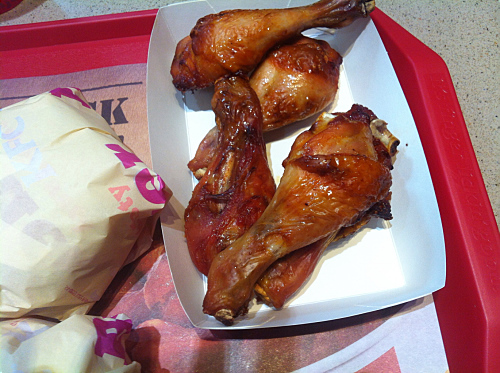In this top-down photograph, we see a red plastic cafeteria tray lined with a paper liner that is slightly visible. The main focus is a small paper boat containing approximately four or five grilled chicken wings, marinated and coated in a delicious-looking dark barbecue sauce. The chicken pieces are grilled to perfection, showcasing a light grilled texture rather than a fried one. To the bottom left of the tray sits what appears to be a wrapped burger, nested in a yellowish-beige wrapper adorned with some pink lettering. Below the tray, a table surface with a salt-and-pepper appearance hints at a fast-food restaurant setting. The vibrant presentation of this meal, consisting of juicy grilled chicken wings and a wrapped burger, exemplifies typical fast-food fare.